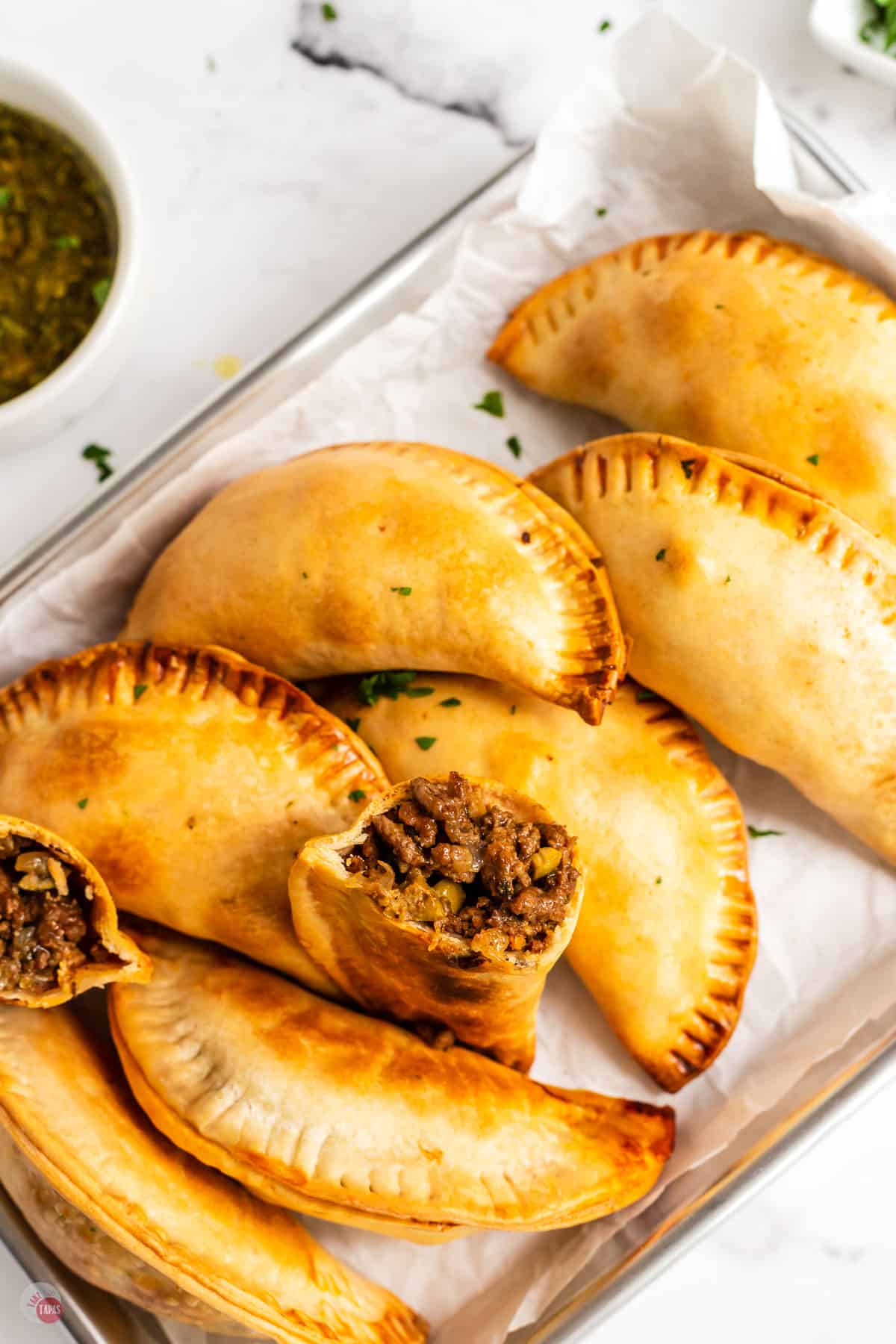This indoor color photograph showcases a silver tray covered with a white napkin, laden with eight golden-brown empanadas, some with visible charring on the edges. Six of the empanadas are whole, exhibiting a distinctive half-moon shape with crimped edges. Two of them are halved, revealing a savory filling of pork, cheese, and possibly beans. The halved empanadas offer a tempting view of their succulent, brown interior. There are two small bowls in the image; the top left features a filling mixture, likely the same meat used in the empanadas, while the top right contains sliced green scallions. The arrangement suggests a cozy, home-cooked setting, possibly taken in someone's kitchen, adding a touch of warmth and authenticity to the scene.